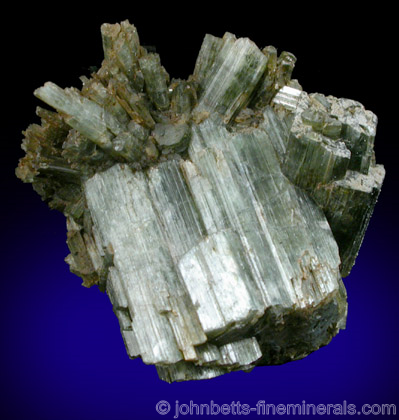This photograph, featured on a website, captures a detailed image of a striking crystal rock formation. The crystal is displayed at a slight angle, appearing as if it is suspended in midair with sharp, rugged edges and intricate internal lines. Its colors range from royal blue, dark blue, and black to silvery-gray, with hints of brown, beige, and a very light green. The background transitions from a predominantly black at the top to blue towards the bottom, highlighting the crystal's metallic sheen and unique texture. Positioned within a nearly square vertical rectangle, the image contains horizontal text in the lower right corner stating, "© John Betts FineMinerals.com," emphasizing its authenticity and source. The photograph effectively showcases the natural beauty and complexity of the crystal, with severe lines and angular formations jutting out in various directions, giving it an almost otherworldly appearance.